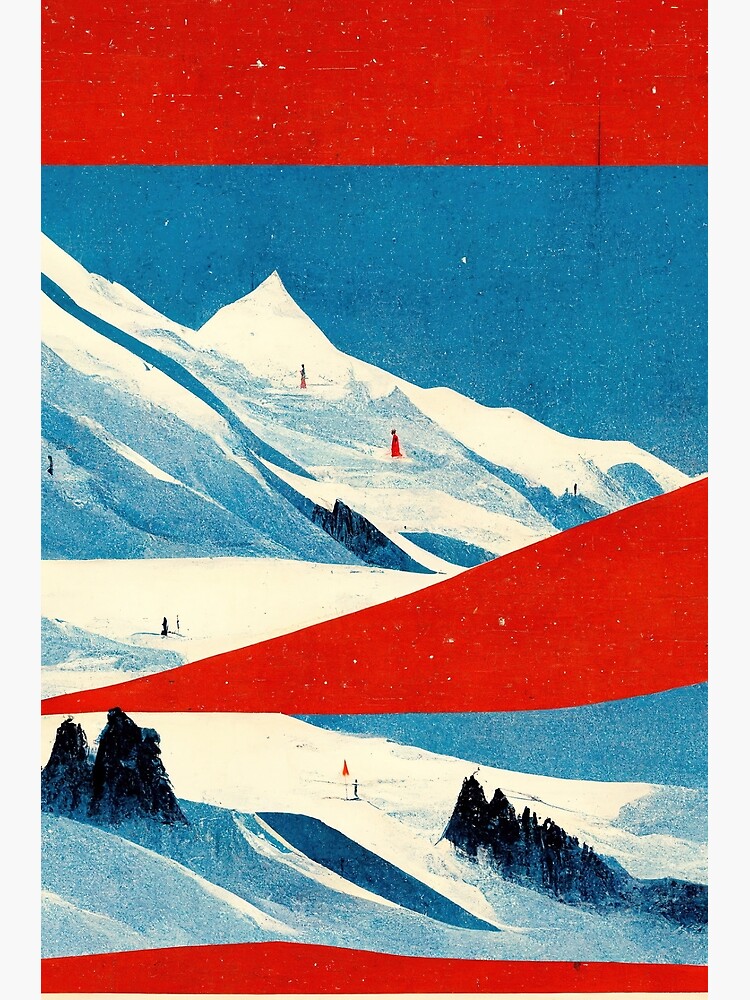This vintage poster, featuring a ski resort scene, shows signs of age and color fading. Encased in a thick white border, the design primarily uses red, white, and blue hues. The top section displays a simplistic drawing with a medium blue sky and white, spiky mountains accented in blue. It shows skiers descending a slope, one in red and another smaller figure higher up. Alongside a red stripe, the sky is dotted with white specks resembling snow. Interspersed on the mountain are red flags, with one or more figures faintly visible nearby due to the distance.

In the middle of the poster, a red band runs horizontally, narrowing on one end and widening conically to the right. This section features a snow-covered landscape with subtle blue shading and a few dark-colored trees.

The bottom part of the poster depicts another level of the hill, accentuated with rolling terrain and more evergreen trees in a greenish-gray tone, set against a blue-shaded snowy background. Here, the red-clad skier reappears along with another skier in black. The poster maintains a simplistic yet detailed style, devoid of any textual elements, focusing solely on the picturesque ski scene.